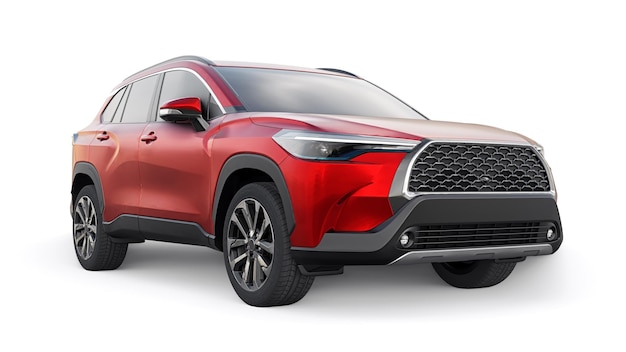The image features a sleek, brand-new red SUV displayed against a pure white background, emphasizing its striking appearance. The SUV, captured from an angle facing slightly to the right, reveals a dynamic 45-degree perspective. It boasts a four-door configuration with silver and black trim, including tinted windows, and a combination of red and black color details. Its grille has a distinct honeycomb pattern with a black, rubber lower section incorporating two circular lights. Notable other features include slim front lights, silver rims, black tires, and a side mirror with a top red and bottom black finish. The roof follows a similar design with black sides and a red middle. Shiny and clean, this red SUV with no visible branding or license plate is styled as though it were photographed for a high-end car brochure.